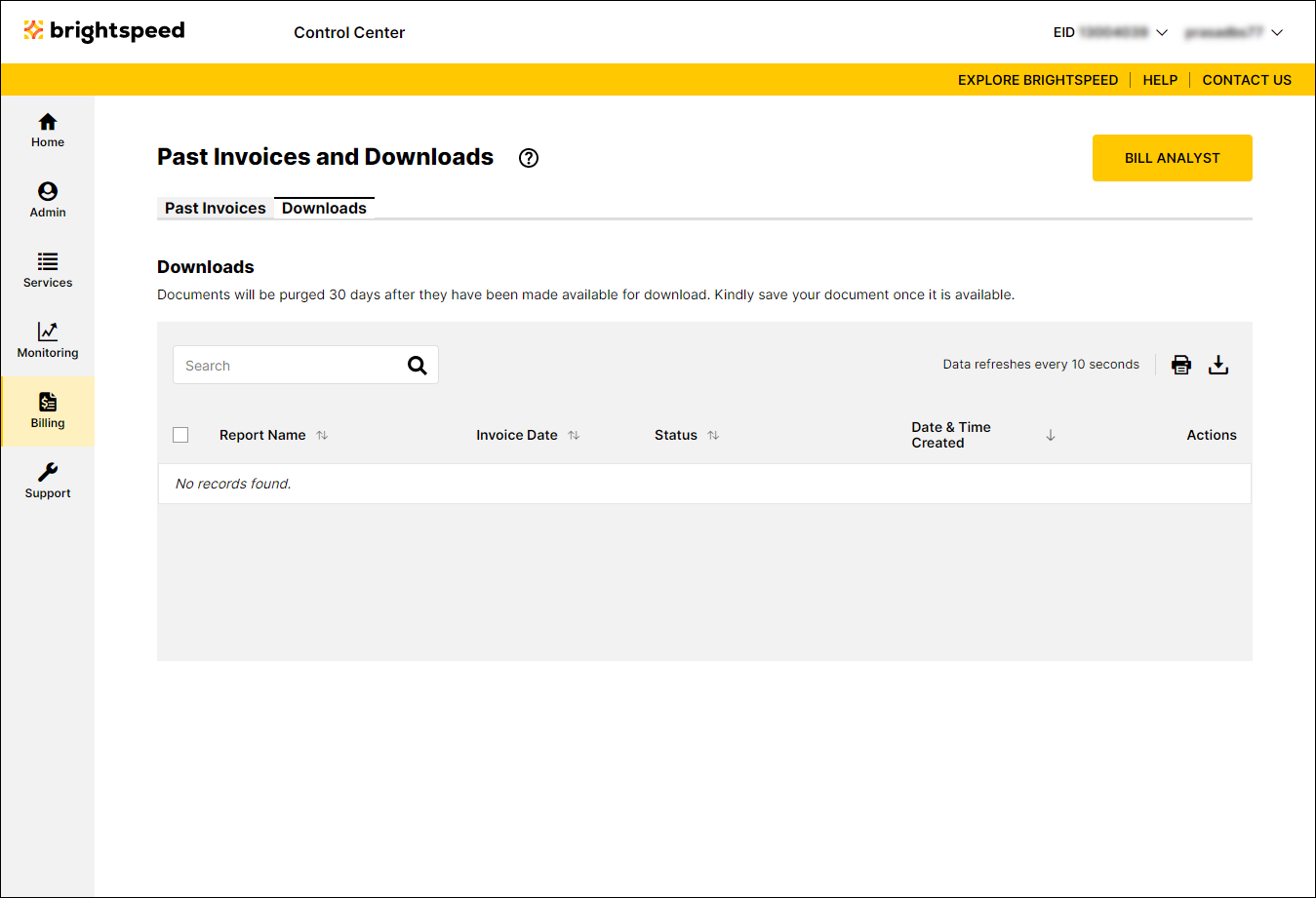In the upper left corner, the word "brightspeed" is displayed in bright, lowercase letters. To its right, the text "control center" is situated. Beneath these words, there's an extended horizontal orange line. Moving further right, options labeled "Explore Brightspeed," "Help," and "Contact Us" are listed.

On the left side, there's a vertical gray rectangle containing a menu with options: "Home," "Admin," "Services," "Monitoring," and highlighted within a yellow box, "Billing." Below this menu, the word "Support" appears, accompanied by an icon of either a wrench or a pair of pliers above it.

Centered in the image are headings "Past Invoices" and "Downloads." To the right, enclosed in an orange rectangle, is the option labeled "Bill Analyst." Below these headings, the word "Downloads" appears, followed by a cautionary note stating, "Documents will be purged 30 days after they have been made available for download. Kindly save your document once it is available."

A search bar with a black magnifying glass icon adjacent to it features below the note. The search criteria listed beneath the search bar include: "Report Name," "Invoice Date," "Status," "Date and Time Created," and "Actions." Above this search area, a message states, "Data refreshes every 10 seconds," with an icon of a printer displayed beside it.